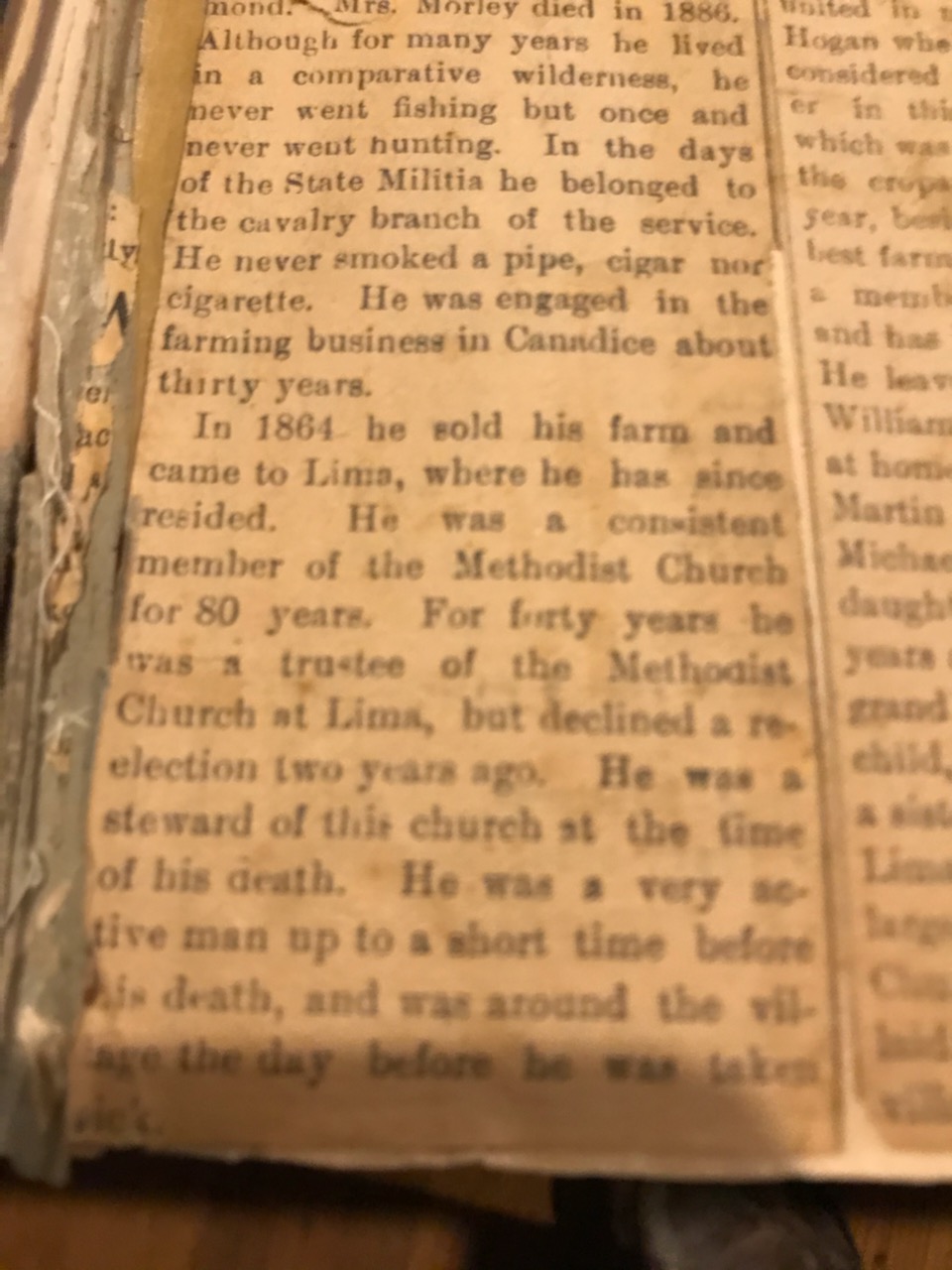This is a slightly blurry, vertically oriented rectangular image of an old, yellowed paper fragment, likely from an old book or news clipping. The left edge of the paper is torn and extra crumpled. The image features black text in multiple paragraphs, although some of the content is cut off or unreadable due to the condition of the paper. The visible text describes an individual who sold his farm in Kansas in 1864 and moved to Lima, where he was an 80-year member and 40-year trustee of the Methodist Church until his passing. The text also mentions that he was a steward of the church at the time of his death and an active man who lived without indulging in smoking or fishing, and only occasionally hunted. The detailed excerpt highlights his engagements in the Methodist Church and his farming background. The visible paragraphs are fragmented, with the text becoming particularly blurry and difficult to read towards the bottom.